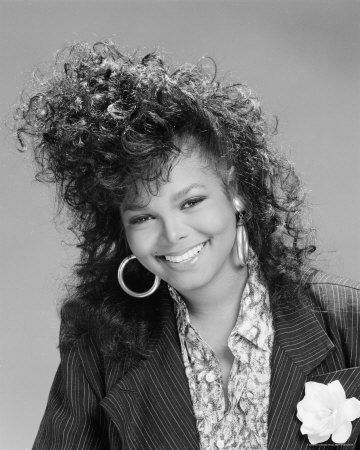This black and white portrait captures a young Janet Jackson with an unmistakable 80s vibe. She is the sole focus of the image, standing against a plain gray background with no extraneous details. Janet's head is slightly tilted to the left as she smiles directly at the camera, her expression warm and engaging. Her voluminous, poofy hair frames her face, a signature style from the 80s. She is adorned with large hoop earrings that dangle near her mouth and wears an outfit that consists of a pinstriped suit coat over a busy patterned button-down shirt. Adding a personal touch, a boutonniere is pinned to the lower right side of her suit coat. The overall composition and her youthful appearance suggest this is an older photo, evoking a timeless elegance reminiscent of classic high school portraits.